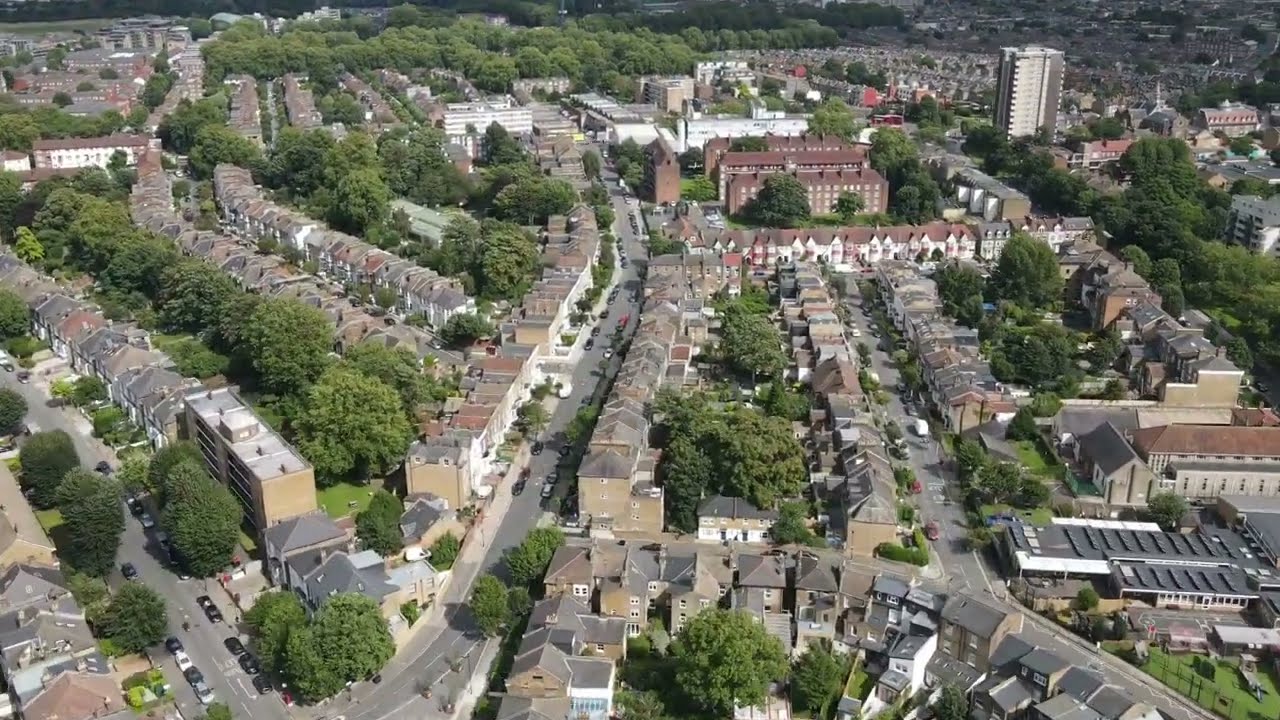This detailed aerial color photograph, taken in landscape orientation, showcases a vibrant cityscape. Central to the image are rows of two to four-story townhomes and smaller buildings, characterized by their brick and grayish-brown triangular roofs. These homes are tightly packed and sectioned into distinct clusters, with streets weaving intricately between them. Adding to the bustling urban feel, numerous tiny cars can be seen moving along these roads. 

A prominent feature slightly to the left is a dark gray asphalt main street that traverses through the center of the image. Toward the top right of this main street stands a large multi-level building with a striking red tile roof, complementing the city’s architectural mix. Nearby, a towering 15 to 20-story high-rise dominates the skyline.

The cityscape is beautifully interspersed with lush green trees that are both among the houses and forming verdant patches in the background, where the urban environment gradually transitions into a more wooded area. This blend of natural and built elements is captured with photographic realism, showcasing the detailed textures and colors from a bird's-eye view provided by drone photography.